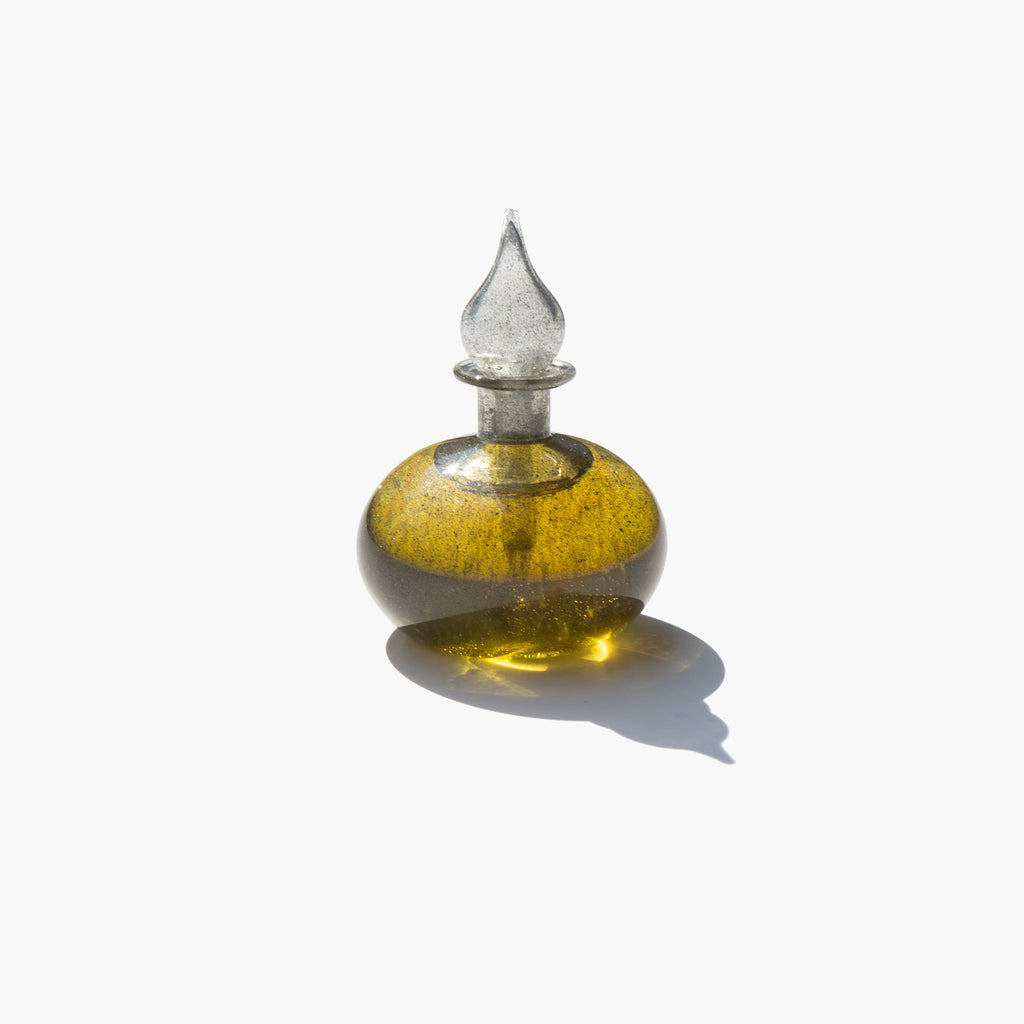The image depicts an elegant, hand-blown glass perfume bottle set against a white background, giving it a floating appearance. The vessel is predominantly spherical, or egg-shaped, with a slender neck. It features a crystal-clear glass dropper styled like a delicate eyedropper or swab, designed to lift and apply the contents. The bottle exhibits a textured, substantially clear glass, hinting at its artisan creation. The liquid inside is a dark, burnt yellow color, suggesting it could be a dense perfume or oil. The top of the stopper is elegantly crafted, teardrop-shaped, adding to the refined aesthetic. The entire piece casts a discernible shadow on the white background, subtly extending toward the viewer and slightly to the east, enhancing its visual depth and highlighting its intricate design.